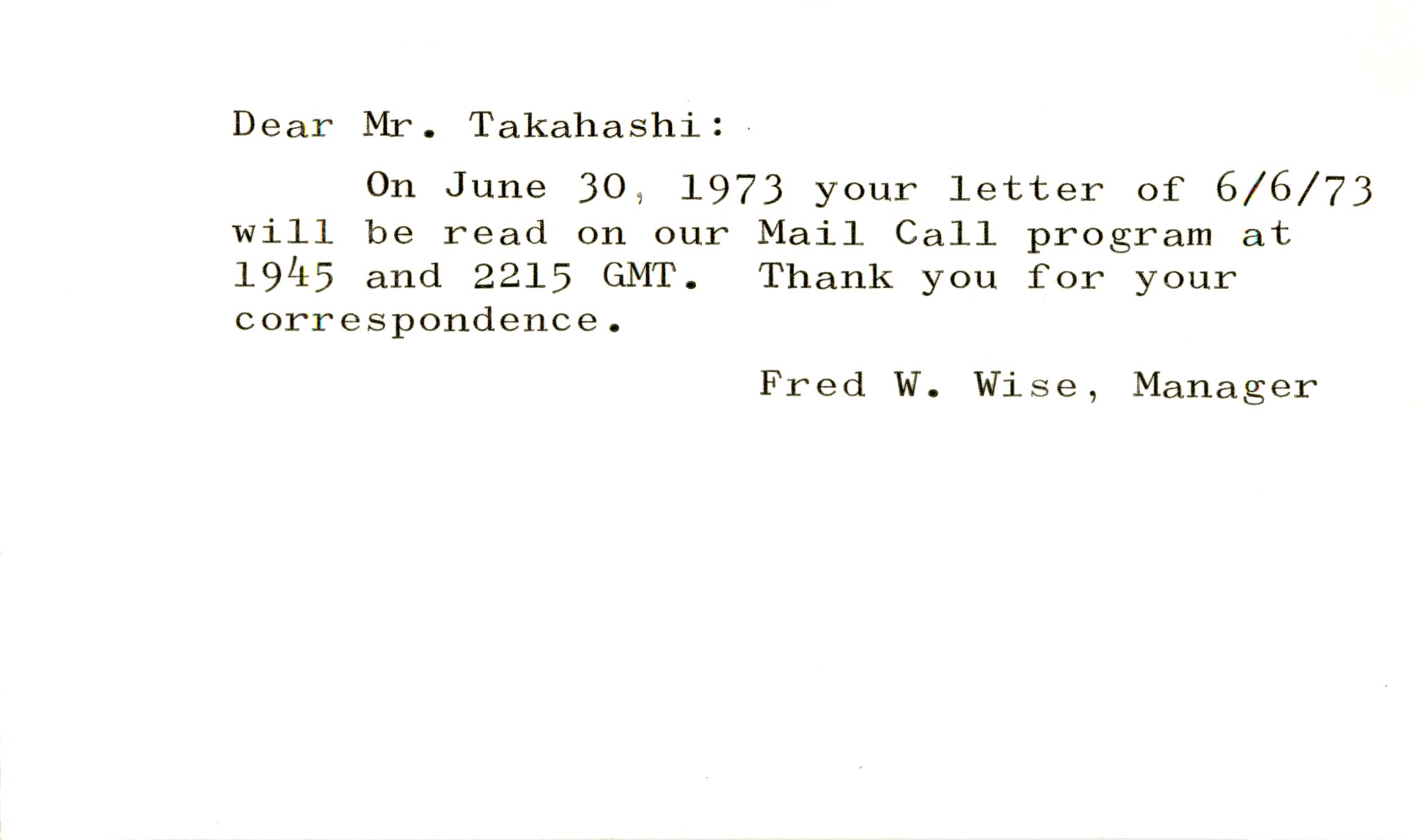The image features a scanned document with a simple, typed letter on a white background. The black text, slightly faded with a subtle yellowish discoloration at the edges, appears to have been typed in an Arial-style font. The letter, addressed to Mr. Takahashi (spelled T-A-K-A-H-A-S-H-I), states: "Dear Mr. Takahashi, On June 30, 1973, your letter of 6-6-73 will be read on our mail call program at 1945 and 2215 GMT. Thank you for your correspondence." It concludes with "Fred W. Weiss, Manager." The layout is straightforward, with small, neat font, giving it the appearance of a professional yet modest correspondence from the year 1973.